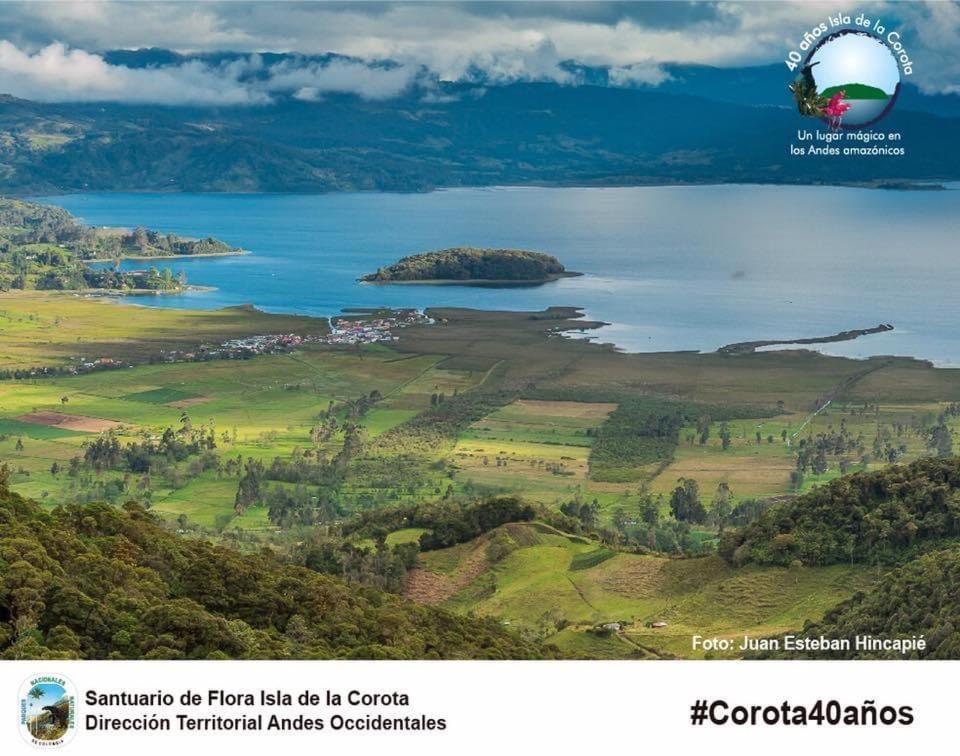This detailed landscape photograph captures a serene and expansive scene, blending natural and text elements harmoniously. At the top, the sky is a deep blue, scattered with white clouds that frame a distant mountain range. Below these majestic peaks, a calm, clear blue body of water likely a lake, reflects the tranquility of the setting. The water's edge meets green fields dotted with varying shades of grasses, some brown patches, and numerous trees and bushes, contributing to the rich tapestry of the landscape.

In the distance, a smaller island stands solitary in the middle of the water, adding a focal point to the expansive vista. Along the coastline, sand can be seen subtly delineating land from water. Towards the horizon, what appears to be white buildings or structures emerge faintly, blending with the surrounding greenery and fields, suggesting human presence amidst nature's vastness.

Overlaying the natural beauty are textual elements: in the upper right-hand corner, white text reads "40 años Isla de la Corota," accompanied by a circular emblem depicting land, sky, and water. Below this, more white text states "Un Lugar Mágico" and "Los Andes Amazónicos." The lower right-hand corner bears the credit "Photo by Juan Esteban Hincapi" in white text, while additional black text is placed at the bottom, grounding the composition with informative and celebratory messages. This comprehensive and evocative image captures the essence and beauty of its natural and cultural elements.